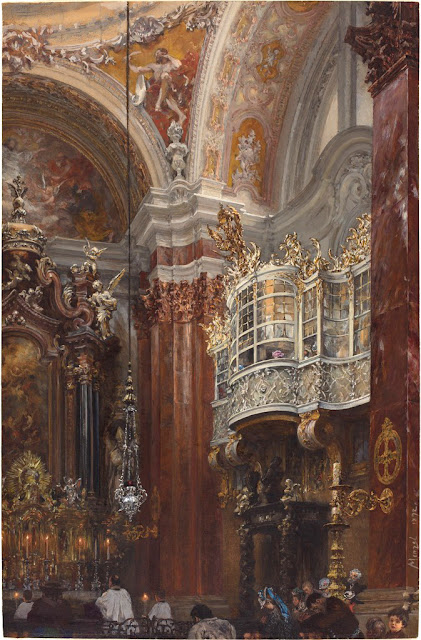The painting depicts a richly detailed interior of a cathedral or church, likely from the Renaissance period, showcasing exquisite and intricate architectural elements that evoke the grandeur of the Vatican City. The scene is filled with notable features, including sprawling archways with ornate white and gold trim, and expansive windows and doors. 

The walls and ceilings are adorned with elaborate paintings and sculptures of angels and heavenly figures, adding to the ethereal ambiance of the space. At the center of the composition, a chandelier hangs majestically, illuminating the setting. 

A prominent balcony, devoid of any individuals, adds depth to the scene, while an altar, equally ornate, stands as a focal point. In front of the altar, two religious figures in robes, possibly priests, are positioned, with lit candles enhancing the solemn atmosphere.

The congregation is visible in the background, seated in pews and observing the proceedings. Notably, a small boy at the bottom right of the painting looks directly at the viewer, adding a personal touch to the grand and holy setting. The painting, executed in oil, encapsulates the opulence and spiritual reverence of a historic cathedral interior.